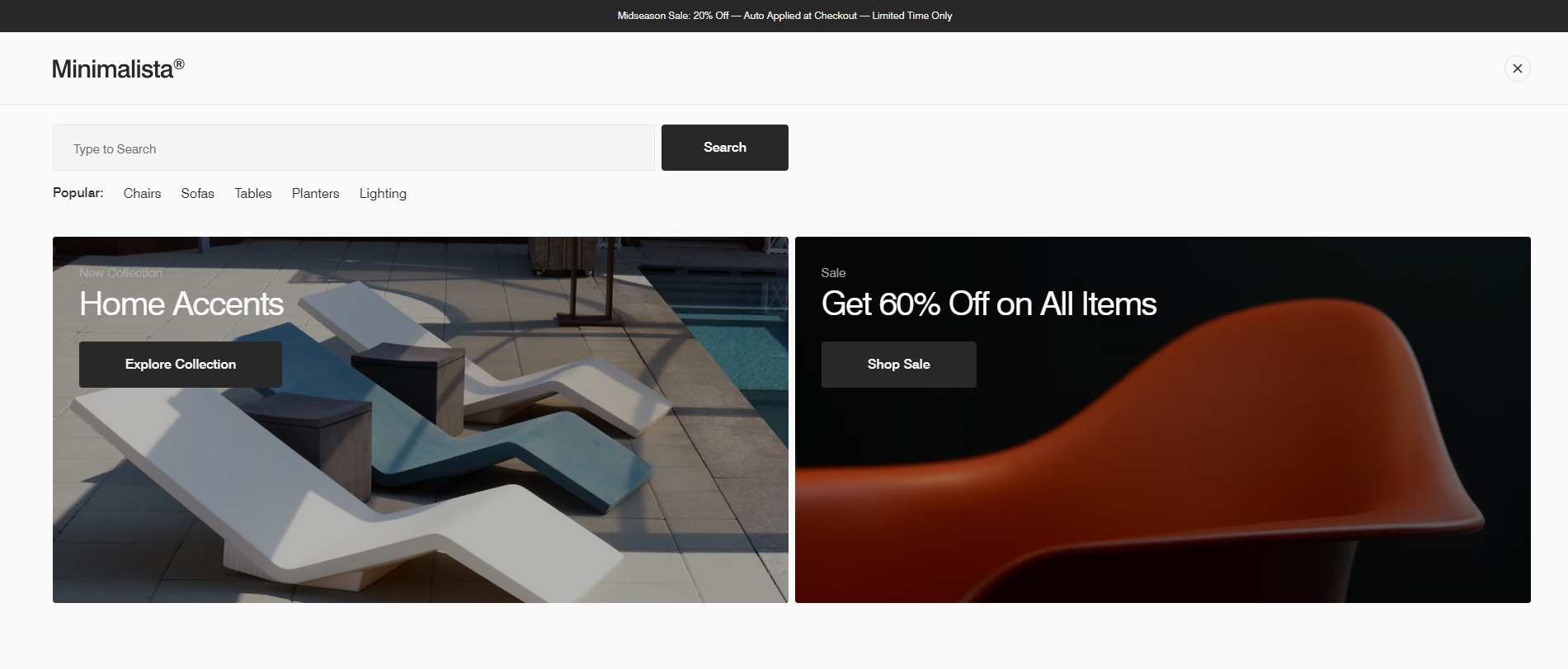The screenshot of the Minimalista website features a sleek, minimalist interface. At the top of the image, a black navigation bar spans across the screen, adorned with small white text in the center, which is unfortunately too tiny to be legible. To the left below this bar, the site’s name, "Minimalista," is prominently displayed. Moving to the top right corner, there is a gray 'X' icon.

Below the "Minimalista" title, a functional search bar invites users to "Type in Refresh or something," accompanied by a black search button labeled "Search" in white letters. Positioned beneath the search bar are navigation text links running left to right, reading "Popular," "Shacks," "Brooks," the rest are unclear but one concludes with "Lightings."

Further down the page, a central image showcases a serene outdoor setting with poolside chairs arranged on a concrete surface near a pool. This section promotes "Home Accents" with the tagline "Explore Collection." Adjacent to this, on a contrasting black background, a promotional image features a striking red object extending from the left side. Overlaying the image, bold white text offers a compelling discount, reading "Get 60% off on all items." Directly below this, a black button with white text urges users to "Shop So."

The overall design of the page is clean and organized, with a focus on high-quality visuals and simple navigation tools to enhance user experience.